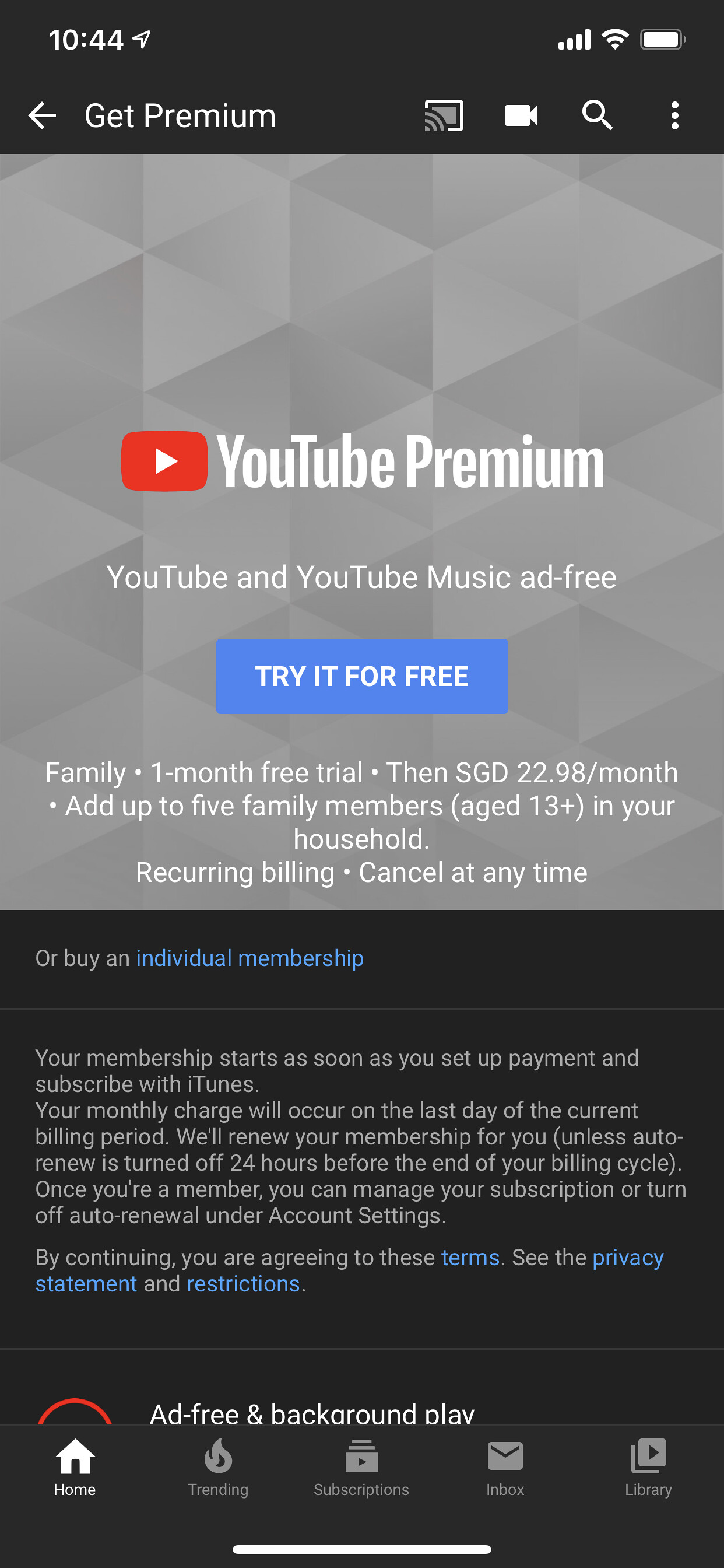This image appears to be an advertisement for YouTube Premium, likely intended for platforms like Facebook. The ad features a sophisticated, grayish geometric background with a black time display showing 10:44, along with several small icons including a search icon.

The central part of the advertisement prominently displays the text "Get Premium" in bold black letters. Below this is the main promotional message "YouTube Premium" written in white font accompanied by a red arrow icon. Underneath, in smaller text, it reads "YouTube and YouTube Music ad-free."

A striking blue box with white text below invites users to "Try It For Free." Directly under this call to action, faint white text describes the promotional offer: "Family one month free trial, then $22.98 a month." It also mentions that users can add up to five family members aged 13 and older within the same household, with recurring billing and an option to cancel at any time.

The middle section of the ad is predominantly black with some blue text, but the font size is too small to read clearly. At the very bottom, the ad features another black strip with white text that highlights features like "Ad-free" and "Background Play." The bottom icons include a home icon and what appears to be an email icon with a partial red circle above it.

Overall, the advertisement is highly detailed and visually structured to promote the compelling benefits of subscribing to YouTube Premium.